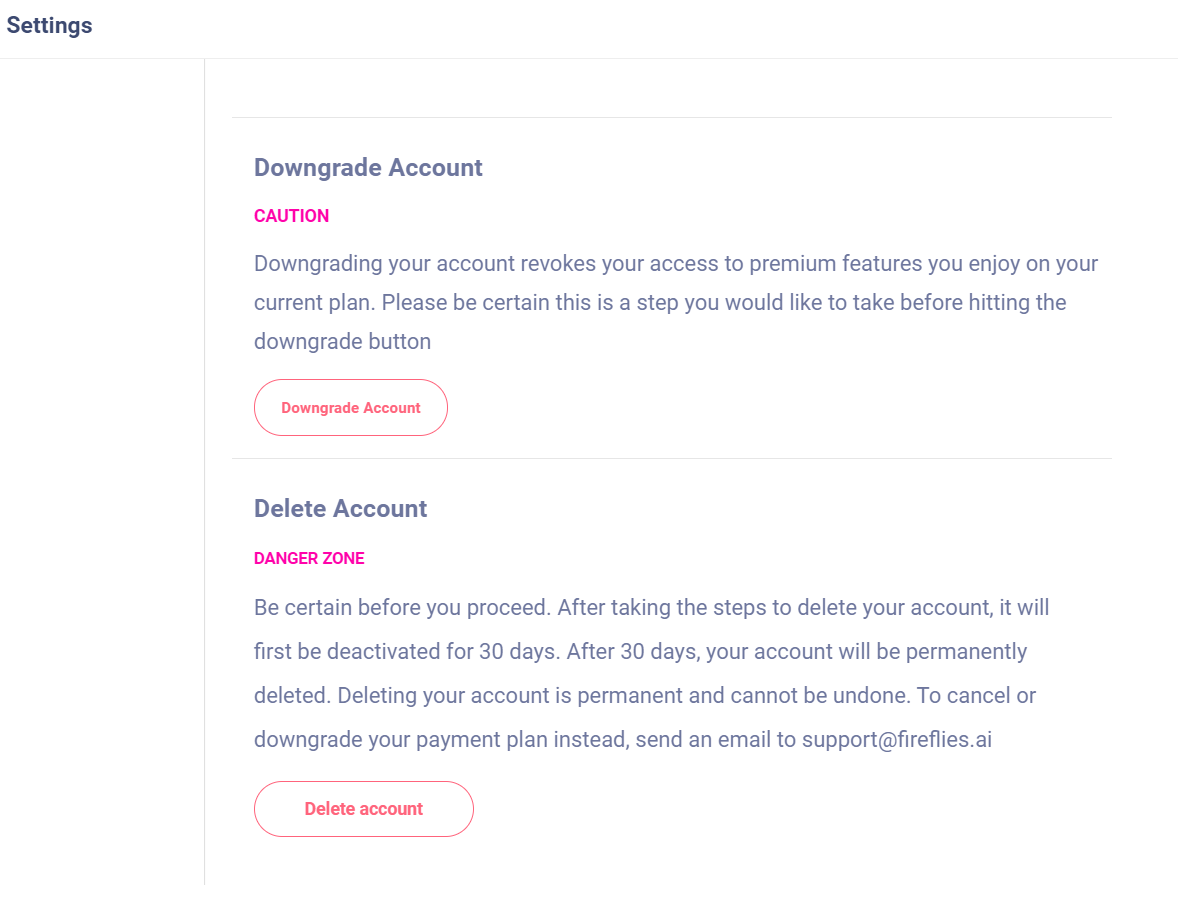The image depicts a user interface screen on a white background with a square shape and a light gray border. At the top left corner, there is bold black text that reads "Settings." Inside the top part of the square, the heading "Downgrade Account" is prominently displayed.

Below this, the word "Caution" is written in purple letters. In gray text underneath, there is a warning message: "Downgrading your account revokes your access to premium features you enjoy on your current plan. Please be certain this is a step you would like to take before hitting the downgrade button."

There is an oblong-shaped button approximately an inch long, matching the background color but outlined with a red border. The button features red text that says "Downgrade Account."

Below the button, a gray horizontal line separates this section from the next. The text "Delete Account" appears in bold, followed by a section labeled "DANGER ZONE" in capital letters with purple text. In gray text below, it cautions: "Be certain before you proceed. After taking steps to delete your account, it will first be deactivated for 30 days. After 30 days, your account will be permanently deleted."